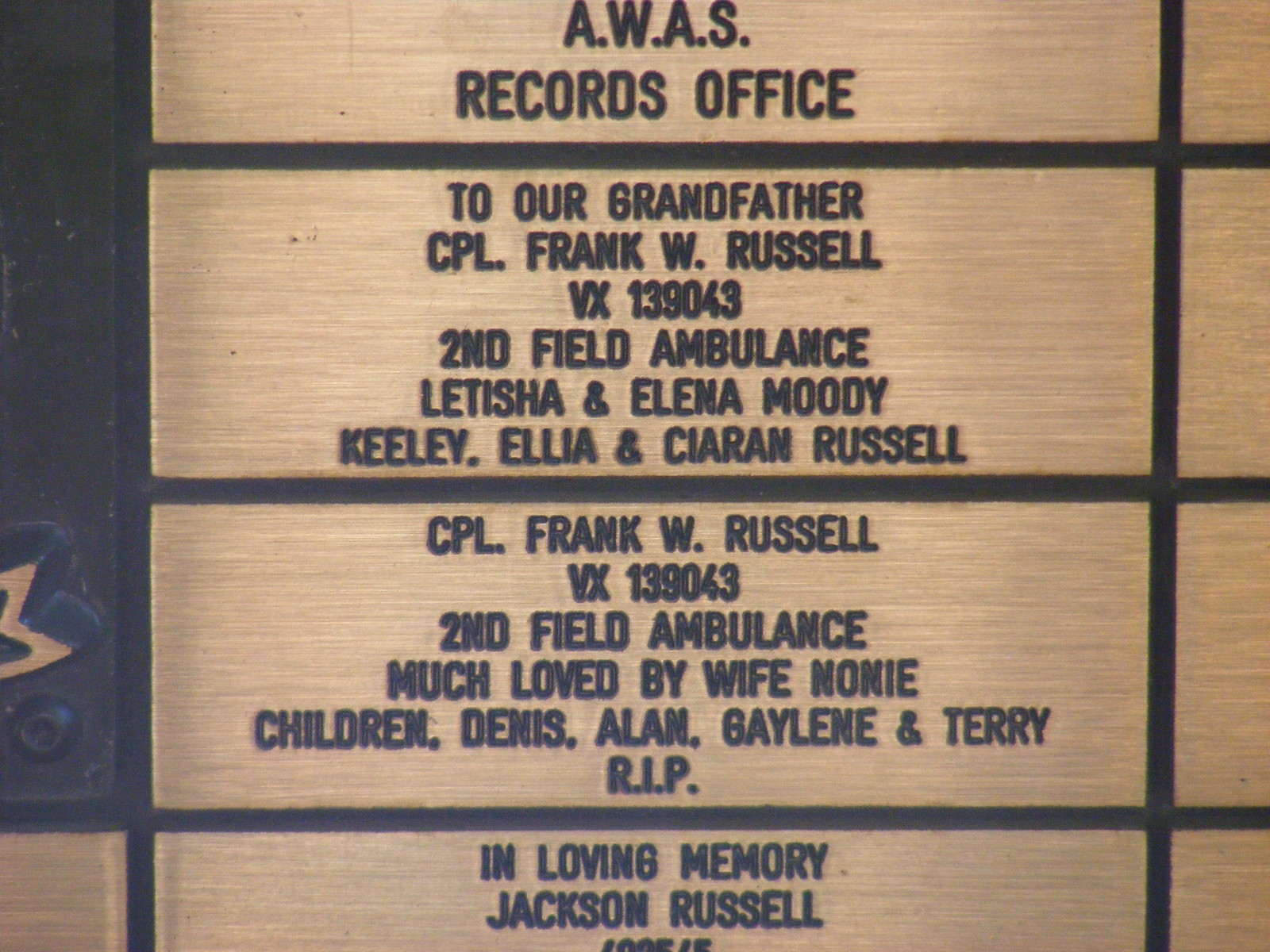This image features a detailed wooden plaque, divided into distinct rectangular sections, with each section bordered by black lines. Only the lower part of the top rectangle is visible, which reads "A.W.A.S. Records Office" in engraved or etched letters on a beige background. The middle rectangle commemorates Corporal Frank W. Russell (VX139043) of the 2nd Field Ambulance and is dedicated "To Our Grandfather," listing Letitia and Elena Moody, Keely, Aaliyah, and Sharon Russell. The third rectangle pays tribute to Corporal Frank W. Russell again, reading "Much Loved by Wife Noni, Children Dennis, Allen, Gaylene, and Terry, R.I.P." The bottom rectangle, partially cut off at the lower edge, states "In Loving Memory, Jackson Russell." To the far left of the plaque is a metallic door featuring an indeterminate gold insignia on its lower part. This plaque appears to serve as a commemorative memorial, possibly situated in a monument or museum dedicated to honoring individuals and families who contributed to war efforts.